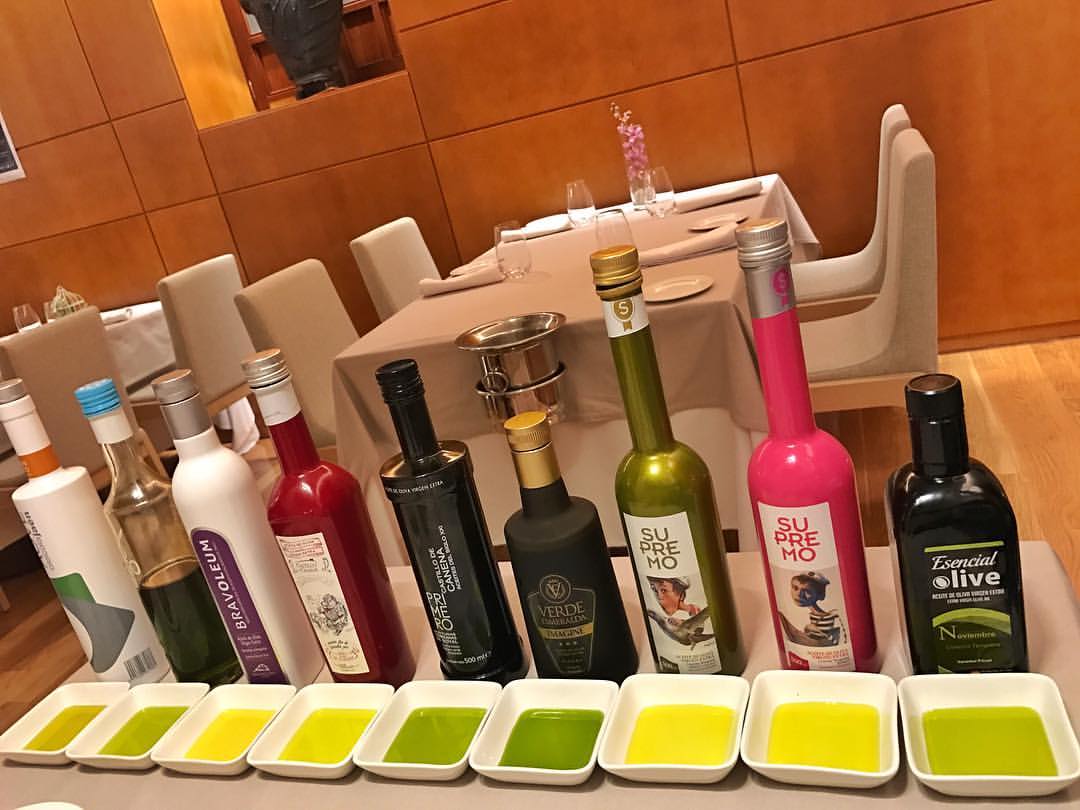The photograph captures the elegant interior of a restaurant, characterized by tables adorned with off-white or beige tablecloths and matching beige chairs with cushioned backs. Each table is meticulously set with rolled-up silverware, small plates, and clear wine glasses. In the foreground, there is a prominent display of nine white ramekin dishes filled with various olive oils, hinting at a tasting session. Behind these ramekins stand an array of sophisticated olive oil bottles, exhibiting a spectrum of designs and colors including black, pink, green, red, white, and clear bottles. Notably, one of the bottles labeled "Essential Olive" suggests a diverse collection of olive oils and possibly vinegars available for tasting. The wall in the background features darker brown paneling arranged in a grid pattern, adding to the restaurant's refined ambiance.